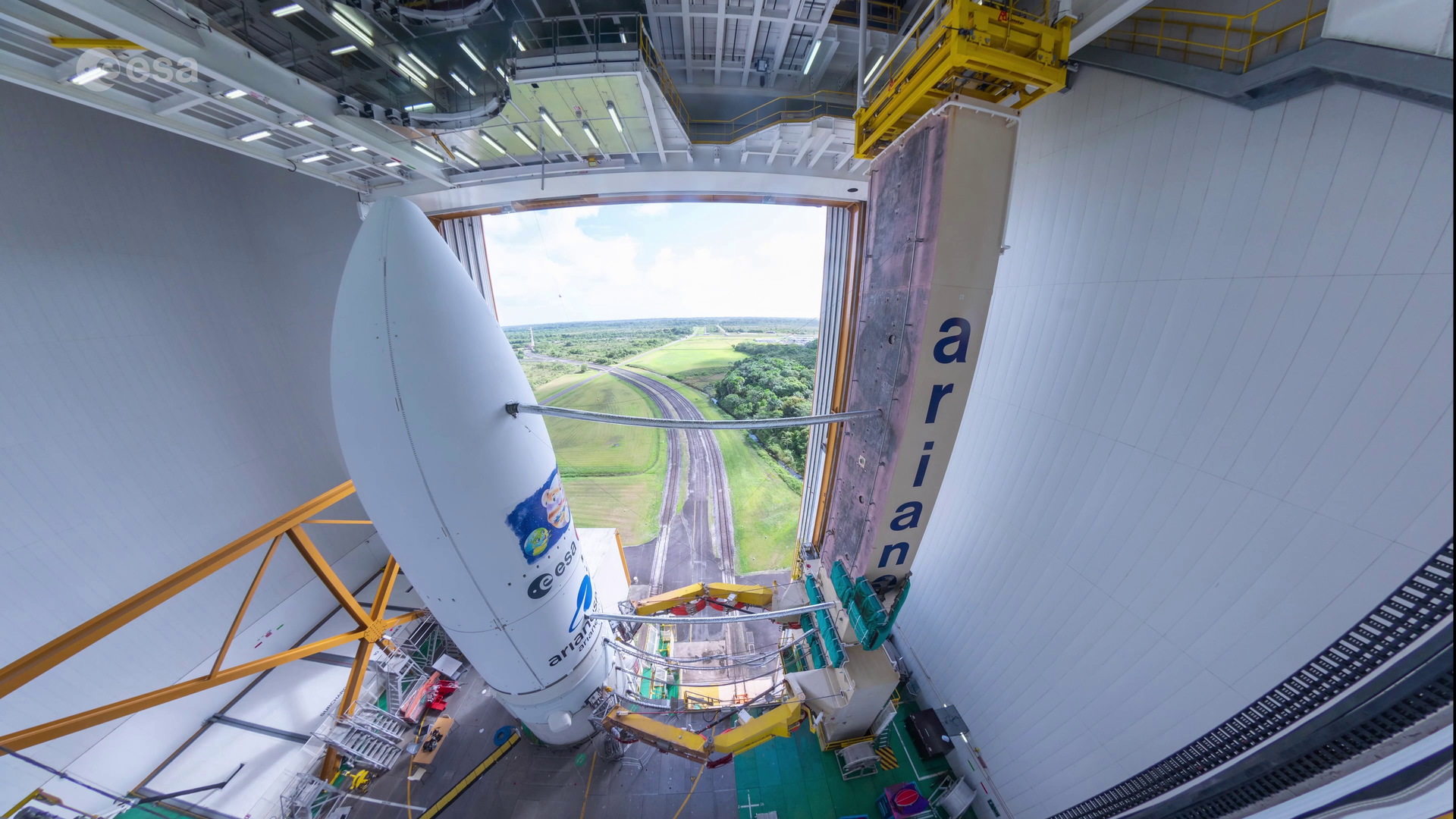This panoramic photograph captures the interior of a vast, open garage-like structure, integral to a space program, likely the Arianne space launch facility. Dominating the scene is a white conical structure resembling a satellite dome designed to sit atop a rocket, bearing the blue letters "E-E-S-A." Adjacent to this, suspended by a yellow grid-like apparatus, is a rectangular block featuring the blue, lowercase letters "A-R-I-A-N." This rectangular block hangs from a well-lit ceiling laced with grid structures. Through the open facade of the building, a curving road is visible, flanked by verdant fields and dark green trees against a backdrop of blue sky and fluffy clouds. This setting indicates the preparation stage for a satellite launch, possibly involving the transfer or installation of the satellite onto the rocket.